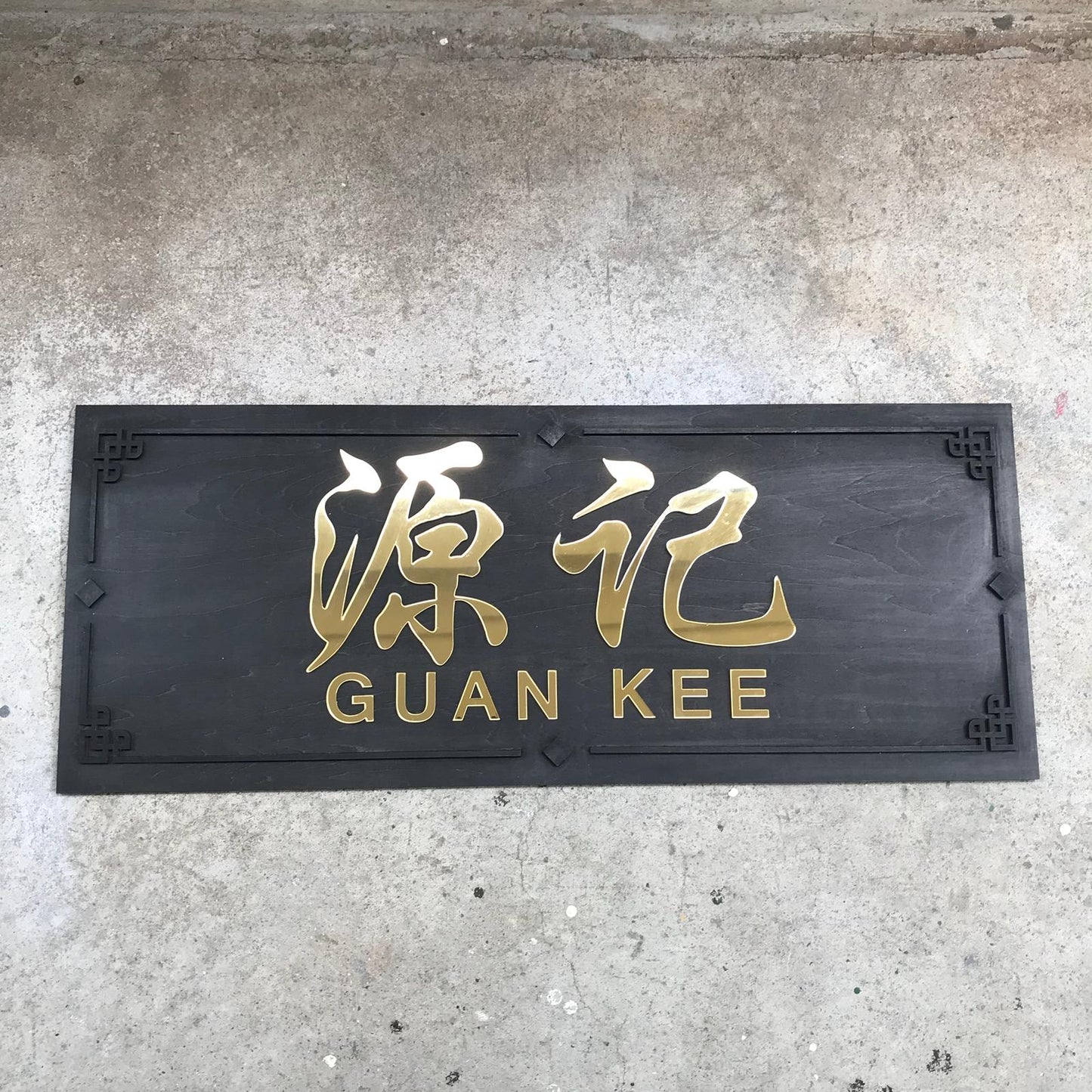The image depicts a rectangular black sign with a darker black ornate border, mounted on a cement or concrete background. The center of the sign is a lighter, grayish-black shade. Displayed prominently in a golden, shiny font are stylized Asian characters, likely Chinese or Japanese, situated above the name "GUAN KEE" in all capital letters. The text is highly reflective, giving off a whitish hue from the light. The sign appears meticulously placed, drawing attention either as a nameplate on a concrete surface or above a restaurant entrance.